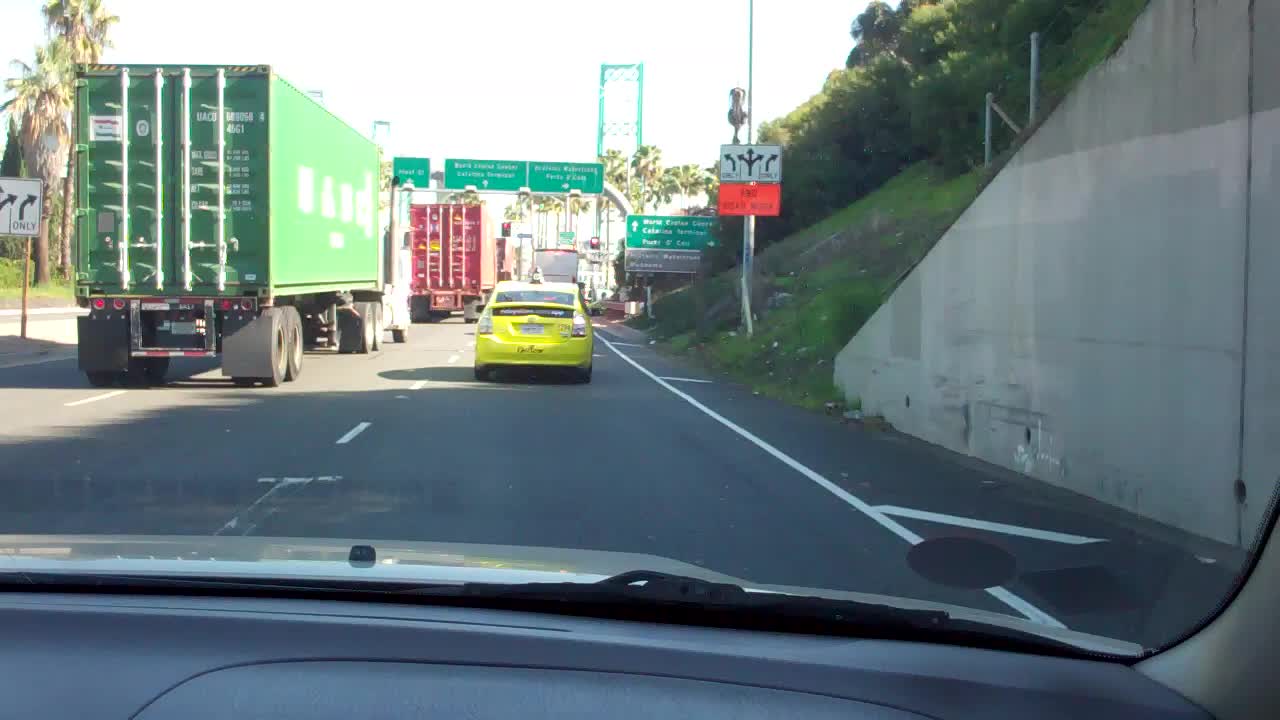The image captures the view through the windshield from the passenger side of a car driving on a two-lane road. A yellow car is visible a few car lengths ahead, traveling in the same lane. Two semi-trucks occupy the left lane, while the concrete wall on the right is angled upward, indicating a hill. Palm trees are noticeable in the background, especially in the top left corner. A road sign mounted on two metal poles is situated in a median, displaying the directive "Turn Only." Additionally, there are three large, rectangular road signs supported by large curved metal poles in the middle background, though the text on these signs is unreadable.